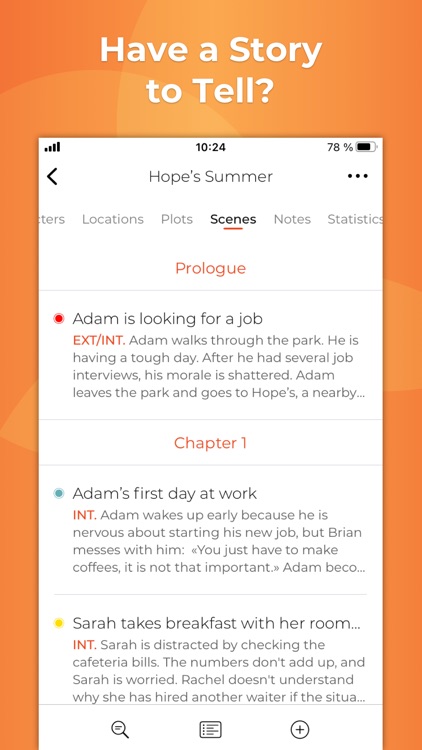Image Description: 

The top of the image features an orange border with the text "Have a story to tell?" Inside the top-right corner, the status indicators show full cellular signal, 70% battery life, and a timestamp of 10:24. The main content is organized in sections that include labels such as "Hope Summer," "Locations," "Plots," and "Scenes," with "Scenes" appearing bolded. The "Statistics" section follows, labeled accordingly.

In red text, a prologue section reads: "Adam is looking for a job. A-X-T-S-H-I-N-T." The narrative begins with "Adam walks through the park; he is having a tough day after losing several jobs. His morale is shattered." Following this, "Adam leaves the park and heads to Hope's nearby."

The image then transitions into Chapter One, again highlighted in red text: "Adam's first day at work." It details how Adam wakes up early due to nerves about starting his new job. The storyline mentions a character named Brian who messes up an inconsequential task like making coffee. Sarah is noted for taking breaks and being distracted by checking cafeteria bills that don't add up. Rachel is confused about her purpose at the job, adding another layer of complexity to the scene.

Icons at the bottom include a magnifying glass, a square, a circle, and a plus sign, followed by the word "white" at the end.